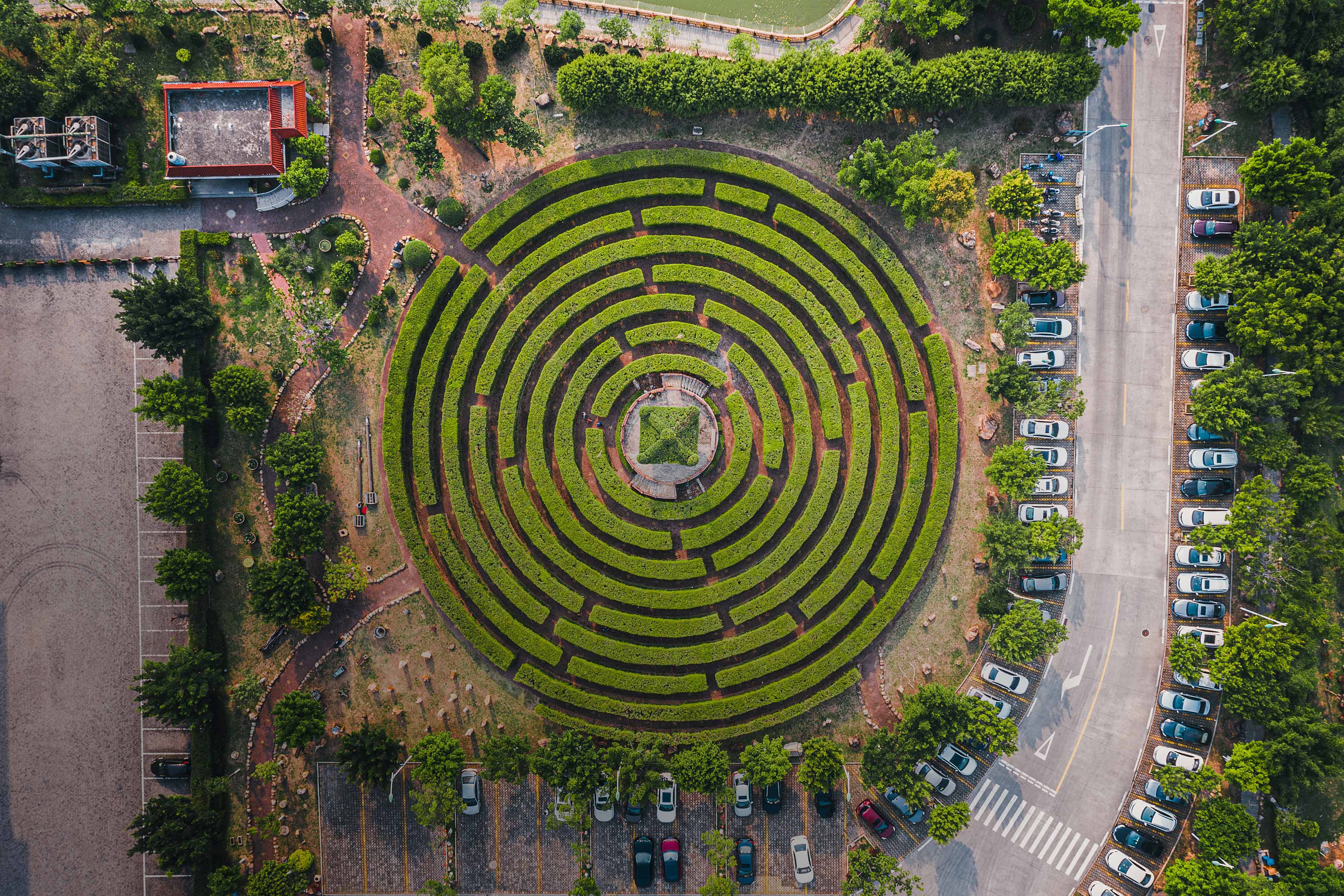An aerial view showcases a large, circular maze meticulously cut into well-kept bushes, nestled in the middle of a city. The intricate design features multiple sections, with openings in the hedges allowing transitions between layers, forming a complex pattern ideal for exploration. Encircling the maze is a reddish clay pathway, adding contrast to the greenery. Surrounding this central feature, abundant green trees create a natural perimeter. To the right of the maze, a busy street lined with numerous parked cars can be seen. On the left lies a patch of concrete accompanied by two buildings, one characterized by a distinctive red rooftop. At the base, there is a parking lot with sparse car presence, while the overhead perspective gives a bird's eye view of the entire structured layout.